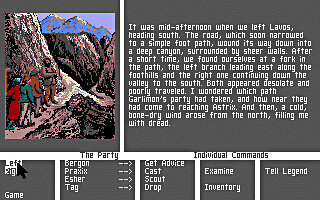This color image is a pixelated screenshot from a retro-style computer game. On the left side, the image titled "The Party" depicts four characters standing on a narrow mountain trail. The background includes towering distant mountains, adding depth to the scene. The pixelated art style gives a nostalgic feel, reminiscent of early video game graphics.

To the right of the pixelated image is a gray text box with a descriptive narrative in white text. The passage details the characters' journey: "It was mid-afternoon when we left Lavos heading south. The road, which soon narrowed to a simple footpath, wound its way down into a deep canyon surrounded by sheer walls. After a short time, we found ourselves at a fork in the path, the left branch leading east along the foothills and the right one continuing down the valley to the south. Both appeared desolate and poorly traveled. I wondered which path Garlamond's party had taken and how near they had come to reaching Asterisk. And then a cold, bone-dry wind arose from the north, filling me with dread."

Below this narrative box are five smaller gray boxes, each containing various types of text, possibly providing additional game information or dialogue.